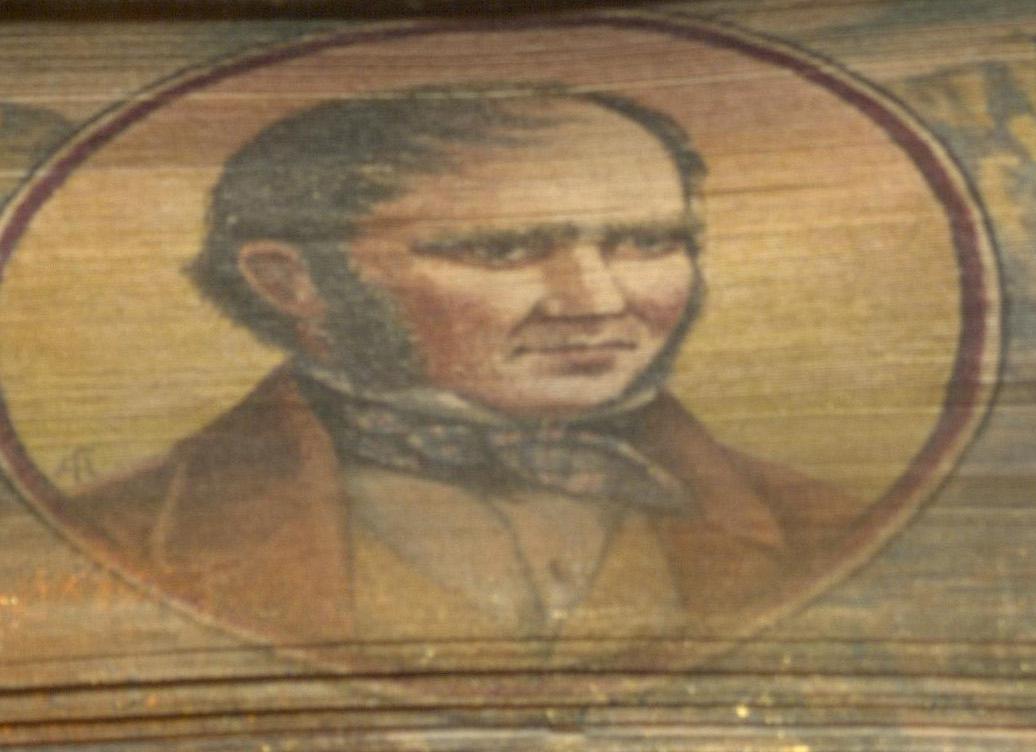This horizontally aligned photograph captures an antique painting on an old wood panel, likely from the 1930s or 1940s. The wood grain, visible through the worn paint, runs left to right. An oval portrait, slightly cropped on the left, dominates the center and is framed by multiple borders: a very thin black outer line, followed by a slightly thicker white stripe, then a mid-width red line, and a yellow background. The portrait depicts a man from the late 1700s or early 1800s, characterized by his balding yet dark, forward-combed hair and prominent sideburns that widen towards his chin. He wears a brownish-tan coat with large lapels, a yellow vest, a white dress shirt, and an ascot-like tie resembling rabbit ears, accentuating his somewhat rosy cheeks and content, wise expression. The bottom eighth of the painting features fine, horizontal grooves, and the top right corner contains blurry yellow letters over a black background, possibly forming a 'W'. The overall appearance, enhanced by the carved lines in the wood, suggests it is a well-preserved antique artifact.